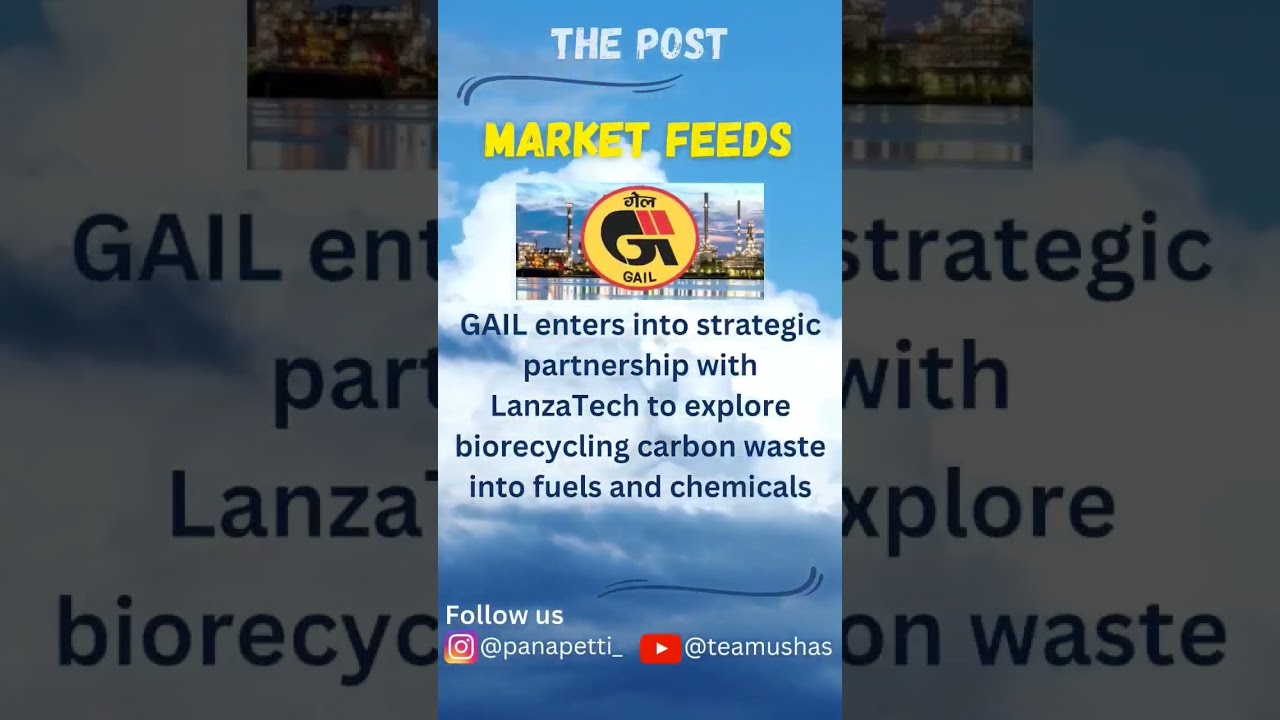The advertisement features a prominent central column flanked by two tinted, darker versions of the same image. The central column, set against a backdrop of clouds, presents a marketing message for GAIL. At the top, in white block letters, it reads "The Post." Beneath is a stylized blue swish and the text "Market Feeds" in yellow. The focal point is a picture featuring a yellow circular decal with a red outline displaying the letter "G" and the acronym "GAIL."

The main content highlights GAIL announcing its strategic partnership with Lanzatec to explore converting biorecycled carbon waste into fuels and chemicals. This text is framed below the primary image, enhancing the narrative of GAIL's environmental innovation. At the bottom of the column is another swish, followed by the call-to-action "Follow us," with social media handles: Instagram @panapetti_ and YouTube @teamUshas. This detailed depiction underscores GAIL's commitment to sustainability and innovative partnerships.